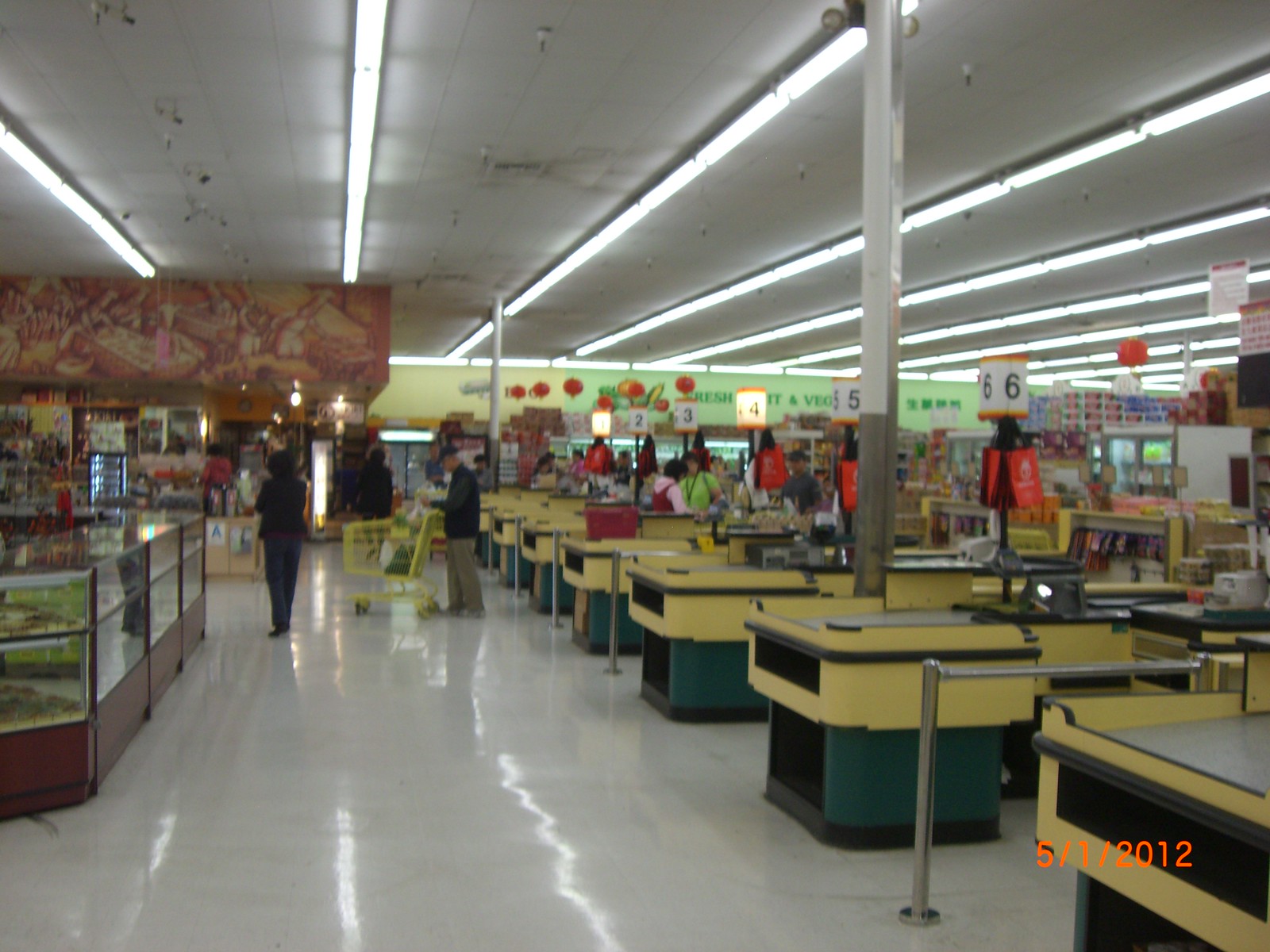The photograph captures a brightly lit supermarket scene, bathed in the glow of numerous fluorescent lights. On the left side of the image, an enclosed glass case stands near a small kiosk, possibly for cigarettes or other small items. A woman dressed in dark clothing walks nearby, while an elderly man, clad in a dark jacket and khaki pants, pushes a yellow shopping cart and appears to be scrutinizing his receipt. Behind them, bins of flowers typically found in grocery stores add a splash of color. The right side of the image is dominated by a row of checkout lanes; only lanes 1 and 4 are open, indicated by the lit-up signs, and customers wait in line. The remaining lanes, marked 2, 3, 5, and 6, stand unmanned. Overhead, strips of fluorescent lighting stretch across the ceiling, ensuring the store is well-illuminated. In the background, the fresh produce section is visible, featuring images of various foods. A date stamp at the bottom of the photograph reads "1 May 2012."